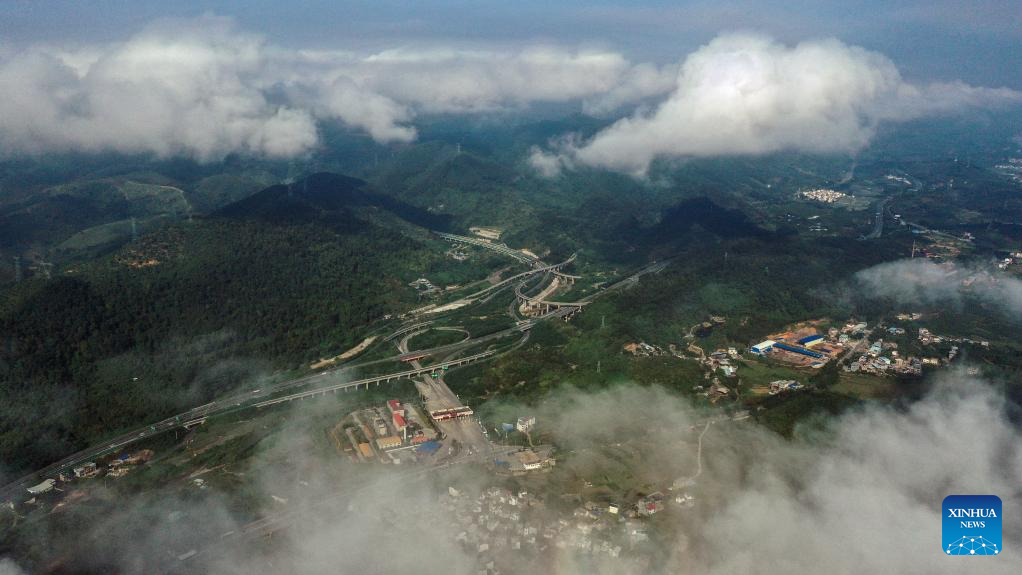This aerial photograph, captured from either a very tall building, helicopter, or plane, provides a breathtaking view of a sprawling landscape that seamlessly blends urban and natural elements. In the foreground, the perspective is high enough to be above the clouds but still low enough to reveal the tops of buildings below. The bottom half of the image displays a network of houses, subdivisions, and shops, intersected by a large interstate system that cuts diagonally from the bottom left corner to the middle, eventually disappearing behind green mountains.

The mountainous backdrop is lush and vividly green, dotted with roads that wind through the hills and connect various parts of the city and suburbs nestled below. The cloud cover is light, casting shadows on the mountains and contributing to a slightly smoky or foggy atmosphere. The urban areas are characterized by a mix of white rooftops and buildings painted in hues of blue and red, creating a colorful patchwork against the natural landscape. In the distance, more mountains and hills can be seen, with additional cities stretched out along the horizon.

A small blue logo in the bottom right corner marks the source of the image as Xinhua News, lending an official touch to this stunning aerial view that captures the intricate tapestry of both urban development and natural beauty.